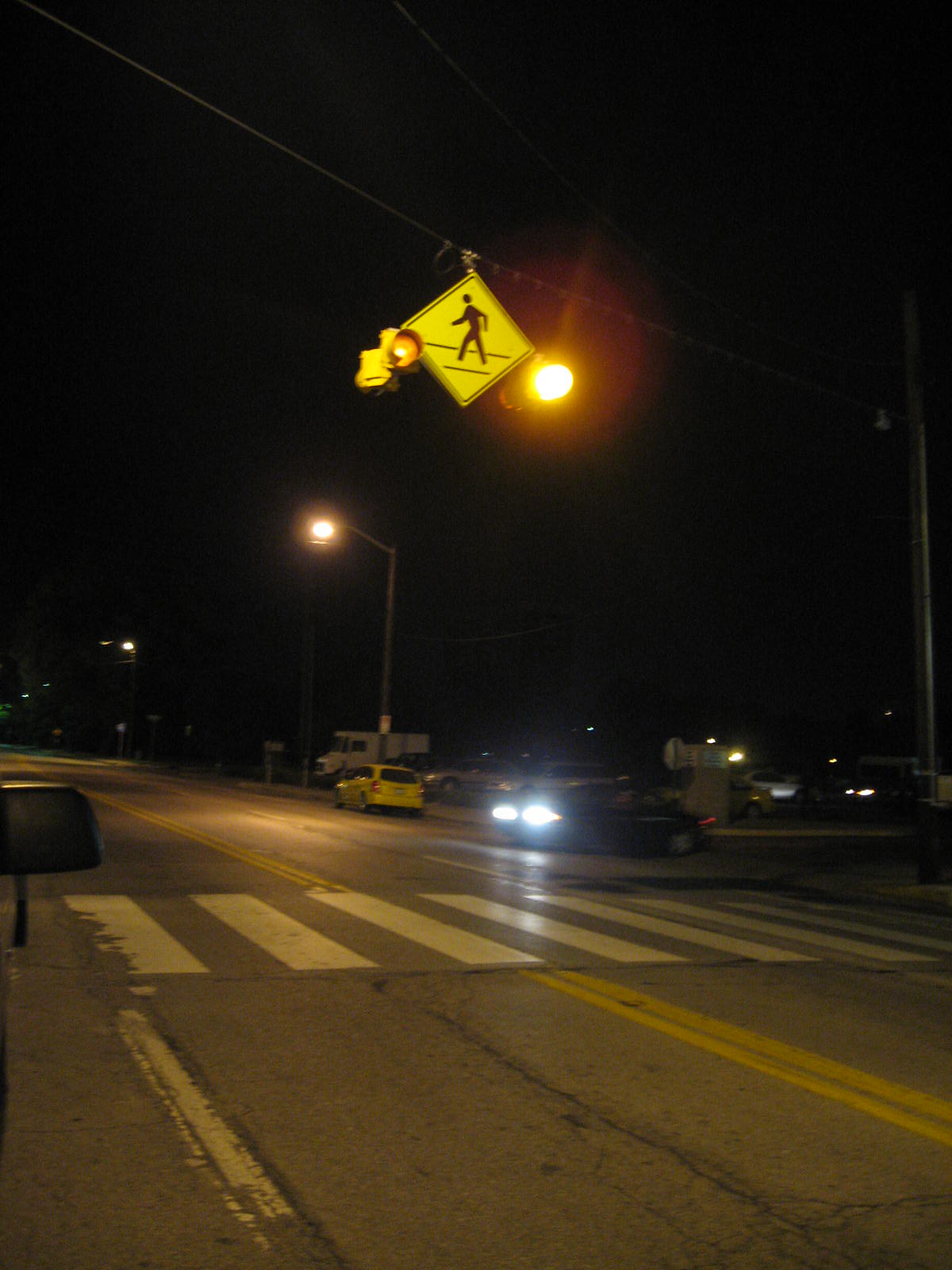In this nighttime color photograph, the pitch-black sky sets a dark backdrop for a somewhat busy scene showcased by the illuminated streetlights and headlights of vehicles. A central element of this image is a crosswalk marked with white stripes and flanked by double yellow lines dividing the road. There is a yellow pedestrian crossing sign with a stick figure symbol, highlighted by two caution lights. The crosswalk spans a road where we can see a yellow car parked along the side, a white truck parked nearby, and another car with its headlights on, moving across the street. The car appears to be emerging from the side, possibly making its way across the crosswalk. While there are no pedestrians visible on the street, the scene also includes some buildings faintly visible in the background and a large parking lot filled with numerous parked cars, suggesting an area with moderate activity despite the absence of people in the immediate frame.